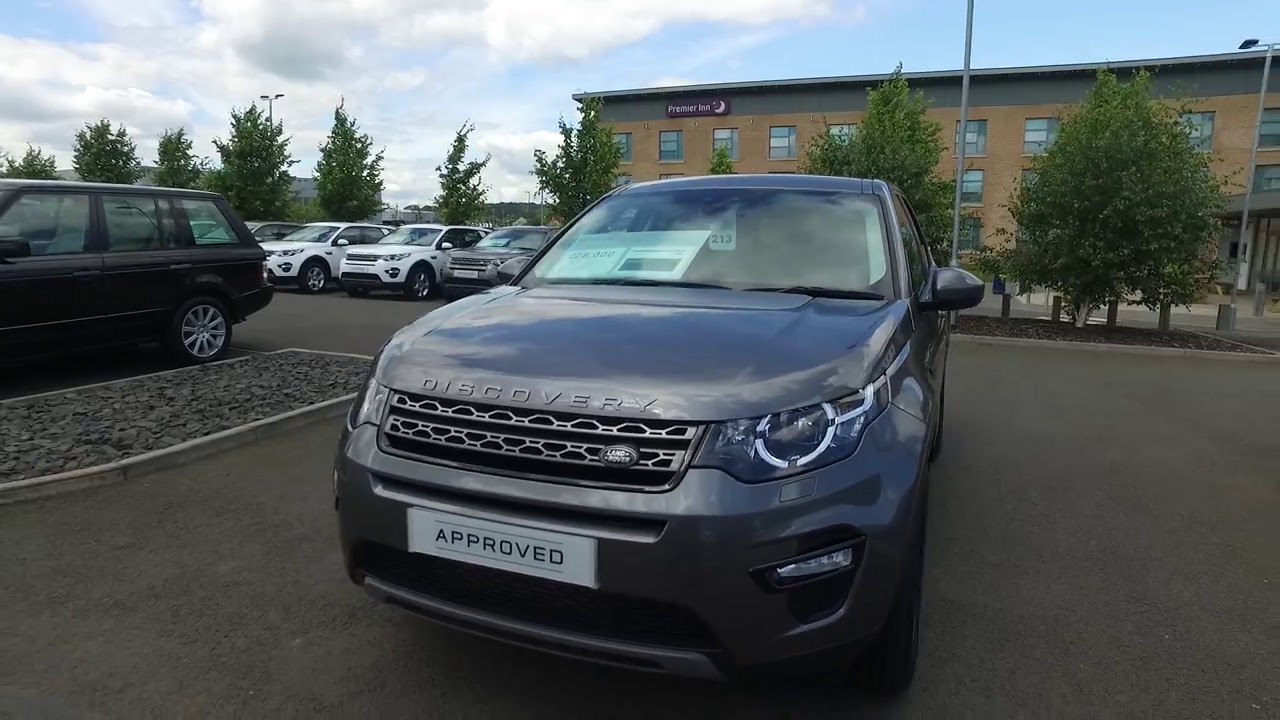This detailed photograph captures a dark gray Land Rover Discovery SUV prominently displayed on a car dealership lot. The SUV features four doors and "Discovery" text on the vehicle, with an "Approved" plate in place of a typical license plate, indicating it is a dealership-approved used vehicle. The front windshield is adorned with various stickers and signs, possibly including the price tag, and has a large sign on the left-hand side. Additionally, the number 213 is visible, hanging from the dashboard. Surrounding the primary vehicle, a variety of other Range Rovers can be seen, including a larger model to its left and additional models in white and blue hues towards the back. The background showcases a substantial three-story brick building with a prominent sign at its top, hinting at the dealership's location. Overall, the scene epitomizes a busy, well-stocked car dealership.